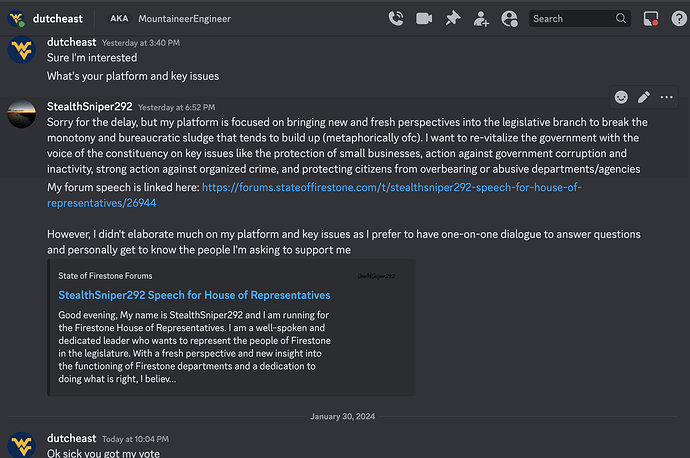A screenshot of a website is displayed, with a primarily black background and white text. The website's information is highlighted in blue. In the upper left-hand corner, the website's logo can be seen featuring a "W" and a "V" stacked one on top of the other against a blue circular background. The owner and poster of the site, "Dutch East aka Mountaineer Engineer," is identified prominently. Various functional buttons such as call, camera, pin, join, and search are present.

At 3:40 PM yesterday, Dutch East posted a message saying, "Sure, I'm interested. What's your platform and key issues?" In response, a user named "Stealth Sniper 292" with a logo depicting a sunset landscape replied, saying, "Sorry for the delay, but my platform is focused on bringing new and fresh perspectives into the legislative branch to break the monotony and bureaucratic sludge that tends to build up—metaphorically, of course. I want to revitalize the government with the voice of the constituency on key issues like the protection of small businesses," and more. At the bottom of the page, Dutch East responds with, "Okay, you get my vote."